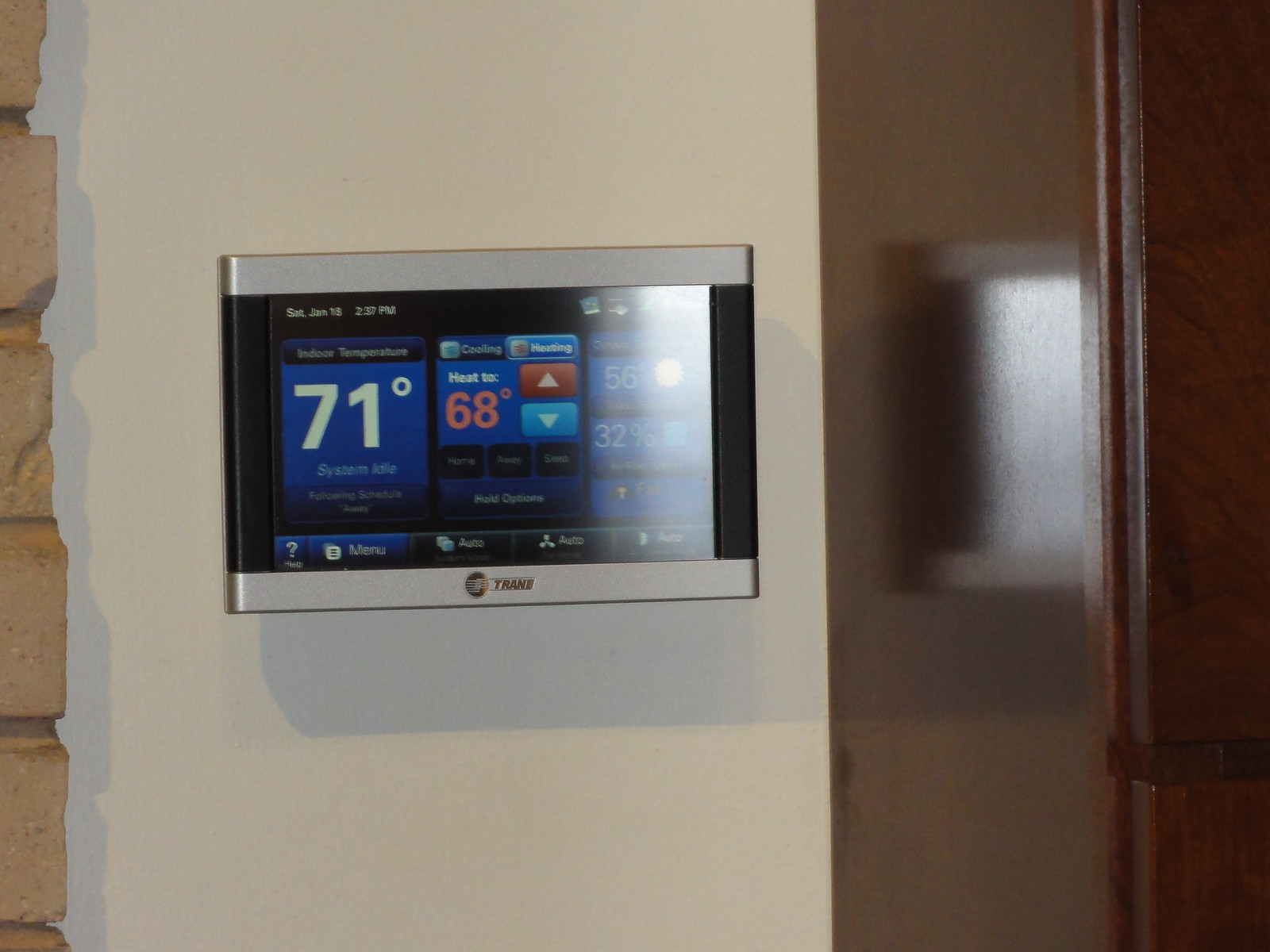On the left half of the image, there is a section of uneven tan-colored brick. Beyond the brick, the shadow casts onto a cream-colored wall. Mounted on the wall is a temperature gauge featuring a metallic silver top and bottom with black bars. The background of the gauge is mostly black, but a light source on the right side partially obscures it. 

The gauge prominently displays a blue box indicating "71 degrees" in yellow text, accompanied by a smaller blue box showing "68 degrees" in red text. Above the "71" box, there is a dark blue rectangle with illegible text. Above the "68" box, there is a smaller rectangle with a greenish square, and another barely readable word. Additionally, beside it, there is a light blue rectangle with an orange spot and some white writing.

The gauge also features a red knob with an arrow pointing upwards, and below it, a blue knob with an arrow pointing downwards. To the right, the wall shifts to a brown color, likely indicating the presence of a window and possibly a door, bordered by wooden elements on the far right side of the image.